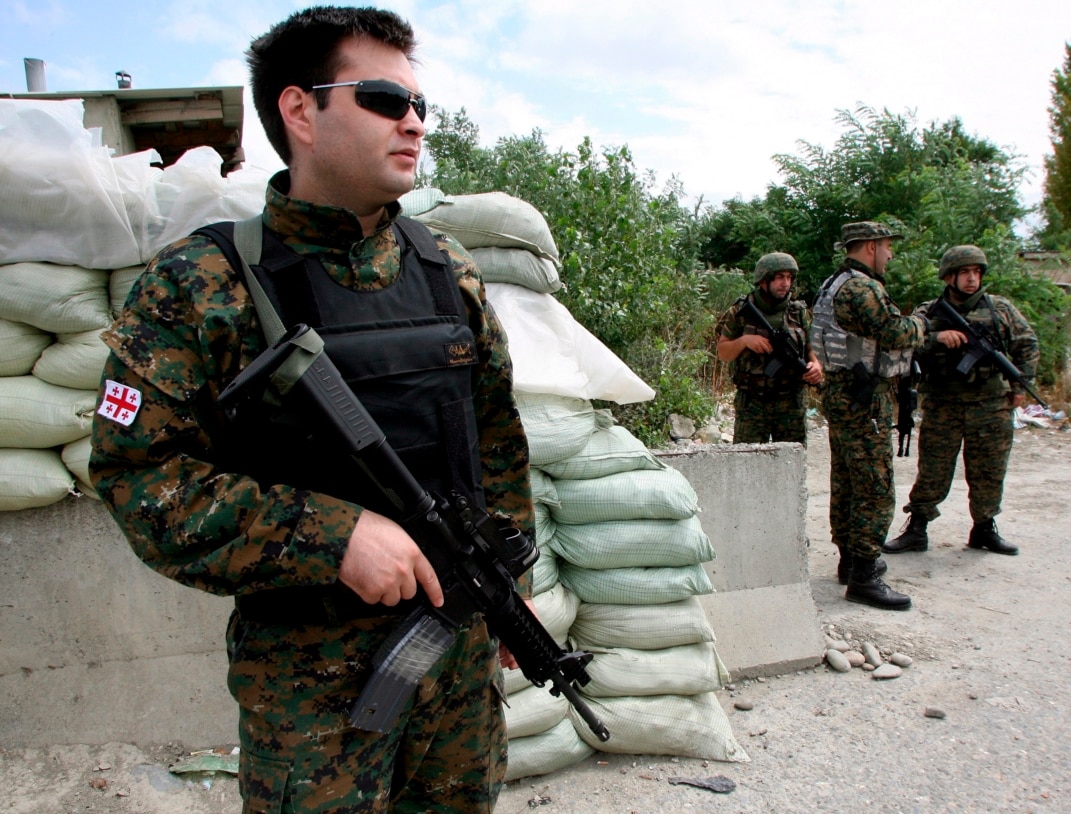The image depicts a group of military personnel set in an outdoor environment with a blue sky adorned by whispery white clouds. In the background, large, leafy trees provide a natural backdrop. In the foreground stands a soldier closest to the camera, wearing sunglasses, with pale skin and short dark hair. He is dressed in green and brown camouflage attire, a black vest with a front pouch, and a notable white flag on his right sleeve marked by a red cross and red dots in the corners. 

He holds a black rifle over his right shoulder, equipped with a green sling and either a clear magazine or tape around it, and is fitted with a black scope. Behind this primary soldier, an arrangement of stacked sandbags forms a makeshift barrier or support structure. To the right side of the image, three additional soldiers stand together, similarly clad in camouflage gear and vests while holding their rifles. Two of these soldiers wear helmets, and one in the middle sports a light gray and white vest along with a baseball-style hat. Near these soldiers, a concrete barrier can be seen. The ground beneath them is a grayish dirt scattered with several rocks.